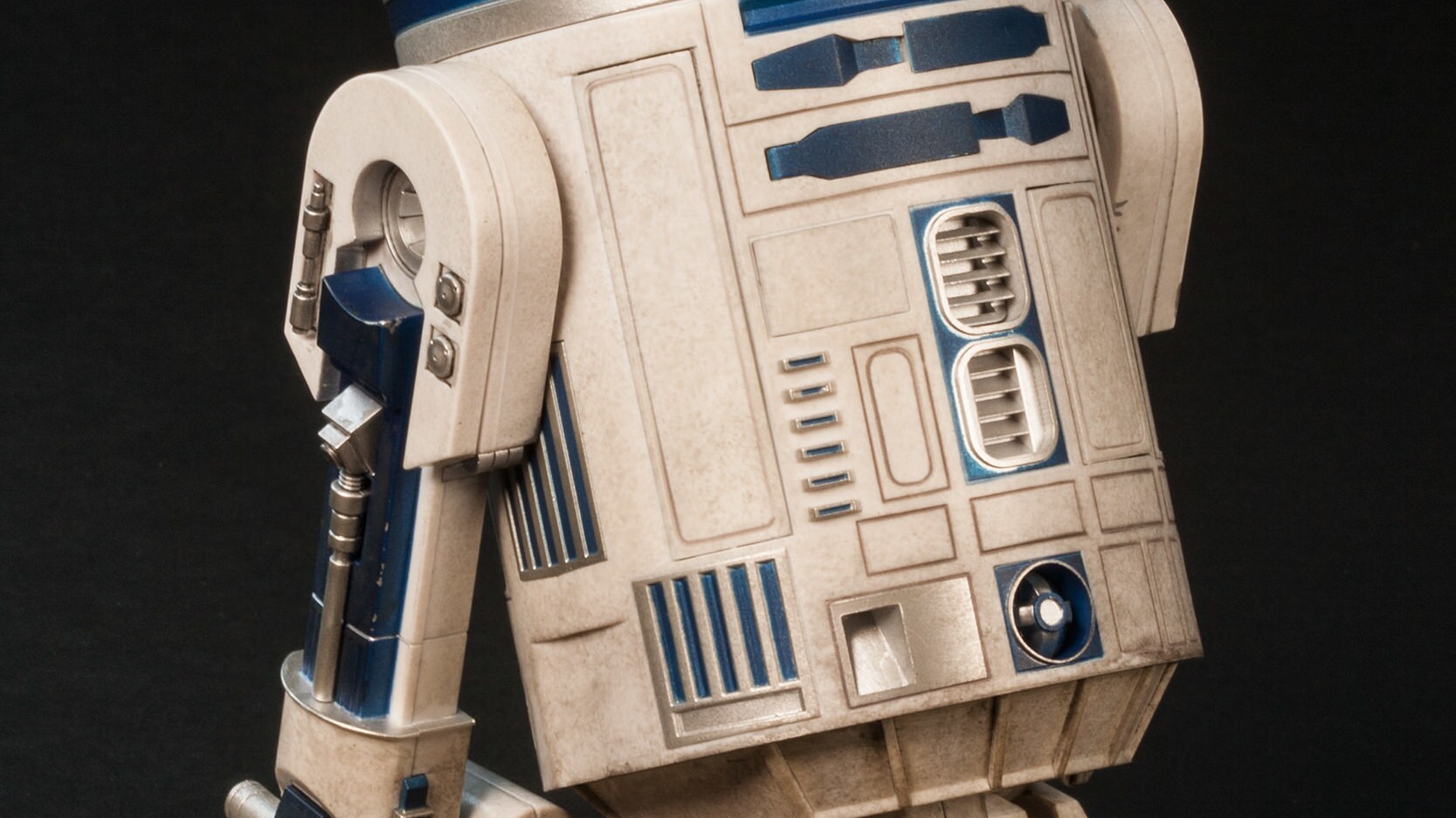This is an up-close photograph of the torso of a robot that closely resembles R2-D2 from the Star Wars movies, possibly fan art. The robot's body is primarily a worn white metal with blue and silver accents, dirtied and weathered from implied use. The figure's detail is highlighted by a stark black background.

Focusing on the torso, the surface is adorned with various mechanical features, including numerous vents, squares, and circular panels, all contributing to its sci-fi aesthetic. Prominent on the upper section of the torso are three horizontal straps, and below them, two vertically aligned silver rectangles with rounded edges and blue backgrounds containing silver lines. Central on the torso is a distinct circle with a white center.

On the left side of the image, a detailed view of the robot’s articulated arm is visible. This arm features a white shoulder joint with silver brackets and blue highlights, adding to the mechanical complexity. Conversely, the right arm is only partially visible, angled away from the viewer, showing just the white shoulder joint. The absence of the top dome and the legs focuses attention on the detailed and intricate torso design.